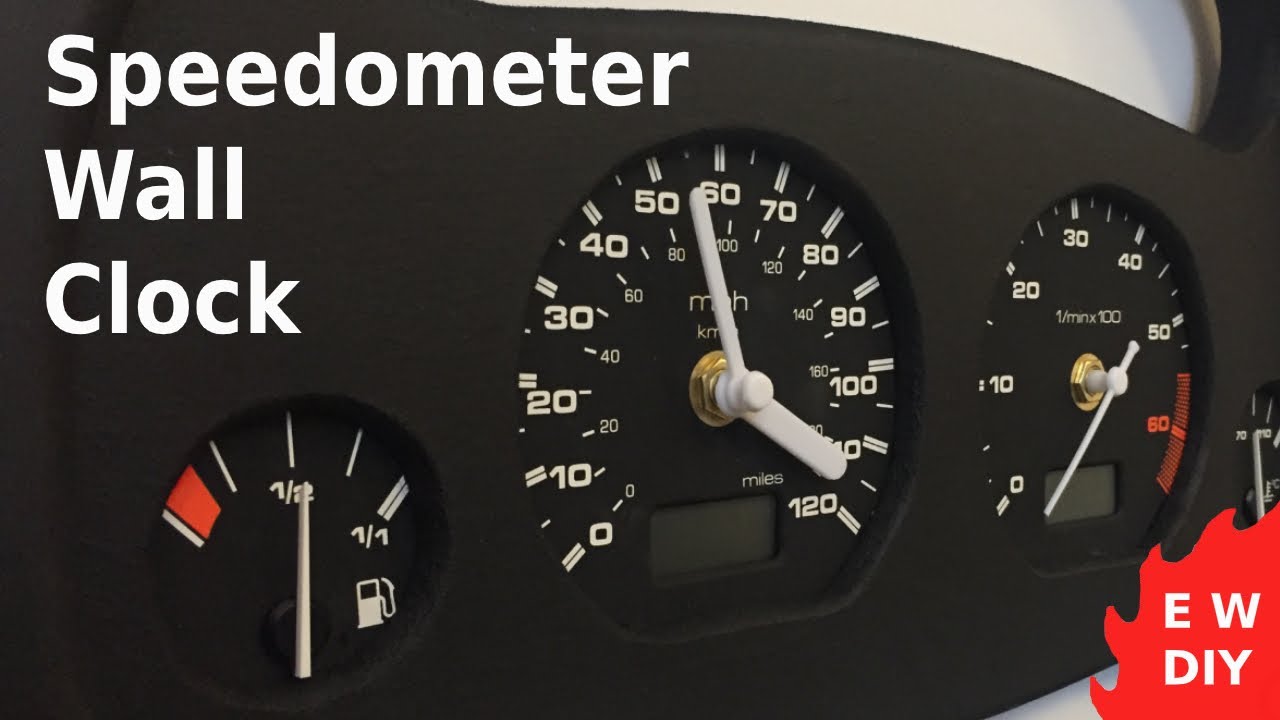This professionally taken, full-color landscape photograph features a detailed image of a wall clock that mimics a car's dashboard. In the upper left corner, bold white text reads "Speedometer Wall Clock," with each word stacked one on top of the other. The clock itself is set against a black background resembling an actual car's dashboard.

The wall clock is black and has three main gauges. To the left is a fuel gauge, showing a half-full reading. In the middle, a large speedometer serves as the main clock face, complete with white hands set to just a couple of minutes before five o'clock. The speedometer dial is marked from 0 to 120, with "miles" written above the 120 mark. On the right side, another round gauge resembles an RPM meter, marked from 0 to 80, with 80 in a red zone. 

In the lower right corner of the photograph, a red flame design encompasses white capital letters spelling "EWDIY." The overall style of the photograph is representational realism, capturing the intricacies and details of the wall clock against its stark, contrasting background.